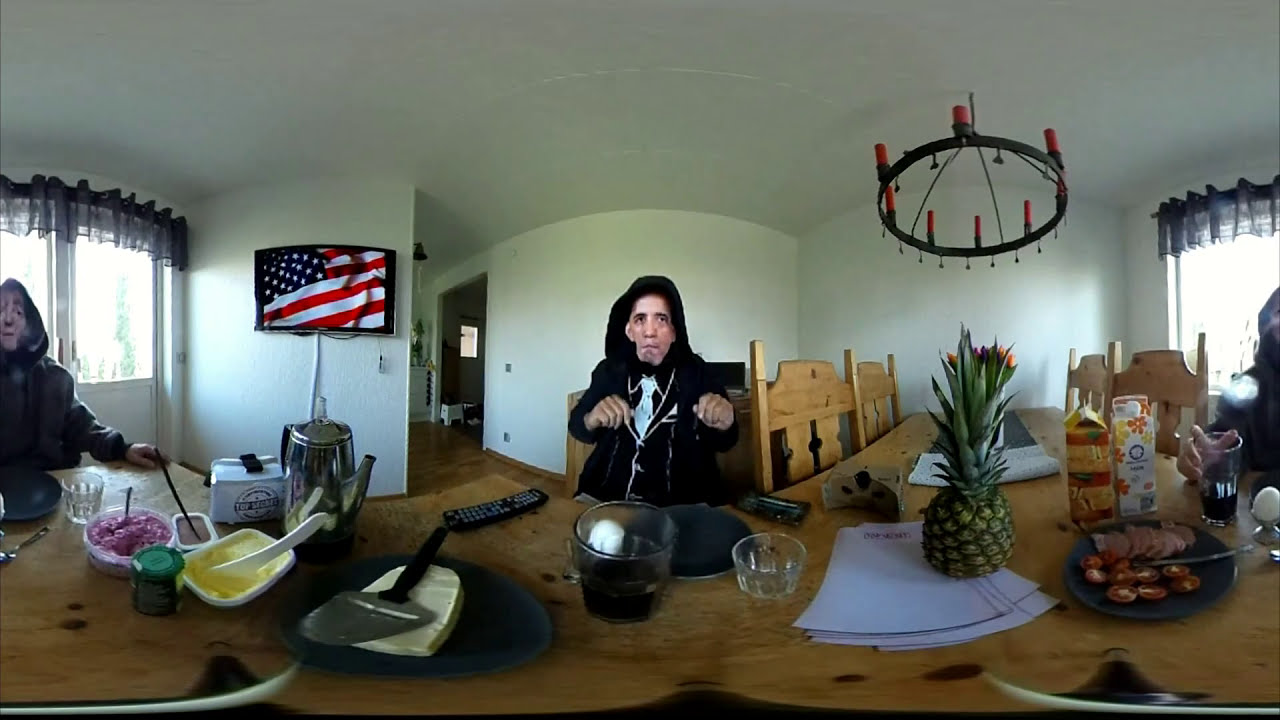This indoor scene captures a dining room with white walls, framed by a window on the left adorned with black valances. A black chandelier with orange, candle-like lights hangs from the ceiling. Centrally, a man wearing a black sweatshirt designed like a faux tuxedo with a white tie and buttons sits at a wooden dining table. The table is scattered with an array of items including an uncut pineapple, several milk cartons, a circular plate with tongs, a glass bowl containing a yellow substance, and another bowl with a pinkish content. A coffee pot and a round tin with a spatula are also seen. Behind him, chairs surround the table. The background features an American flag within a picture frame. The man, with an expression of mild confusion, has his hands raised at chest level, facing the camera.